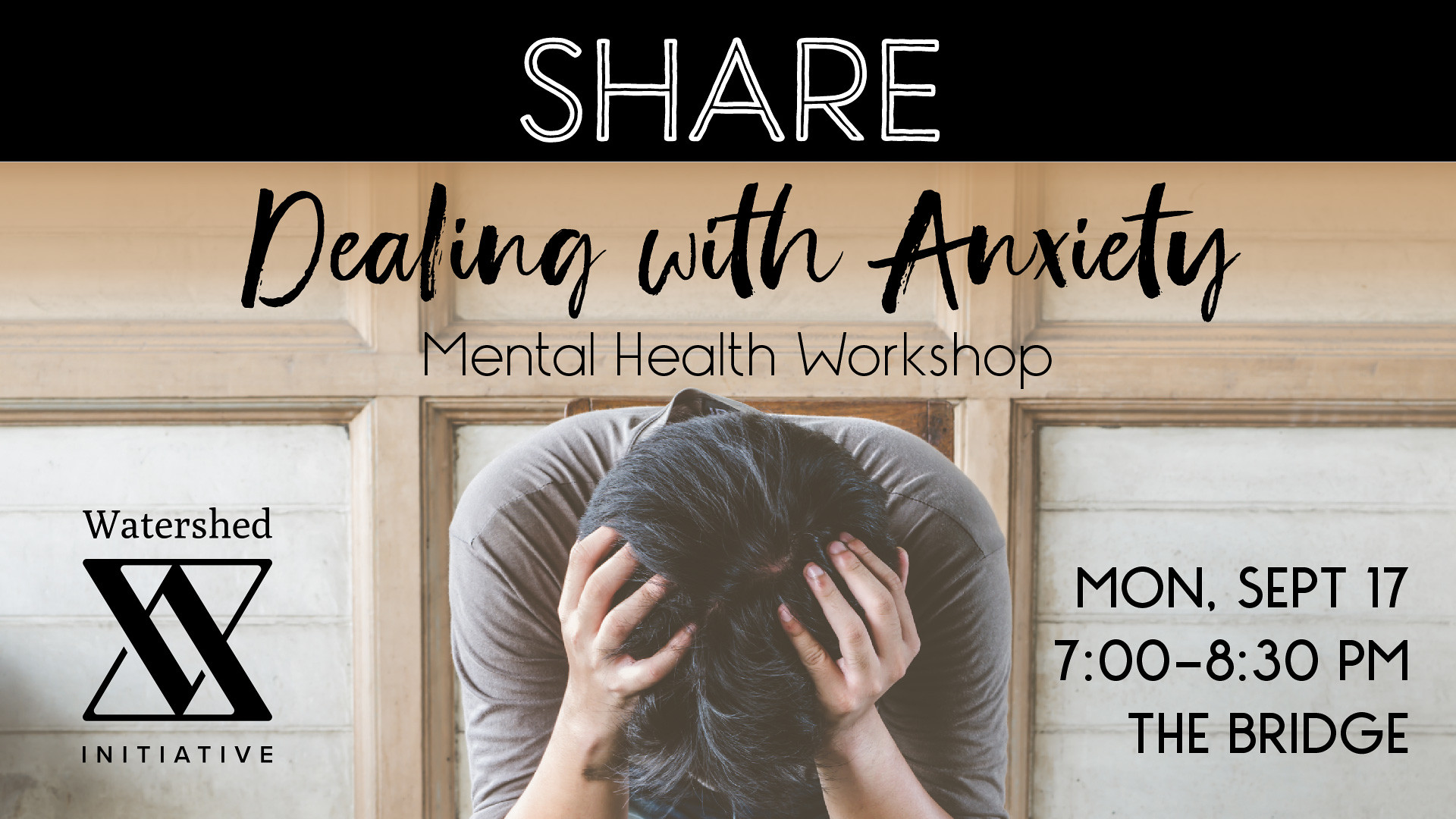This image is an advertisement for a mental health workshop titled "Dealing with Anxiety," which is part of the Watershed Initiative. At the top of the image, a black bar spans from left to right, featuring the word "SHARE" in white letters. Directly below, set against the background of the photo, it reads "Dealing with Anxiety" in cursive script, followed by "Mental Health Workshop" in black letters. The central focus of the image is a person sitting in a wooden chair, wearing a gray t-shirt. The individual has black hair and their head is bowed with their hands supporting it, conveying a sense of frustration or distress. The background features a wooden wall with sections in white and tan. On the lower left of the image, there is the Watershed Initiative’s logo, composed of interlocking triangles, and the name written in black. On the lower right, detailed event information is provided: "Monday, September 17, 7 to 8:30 p.m., The Bridge."